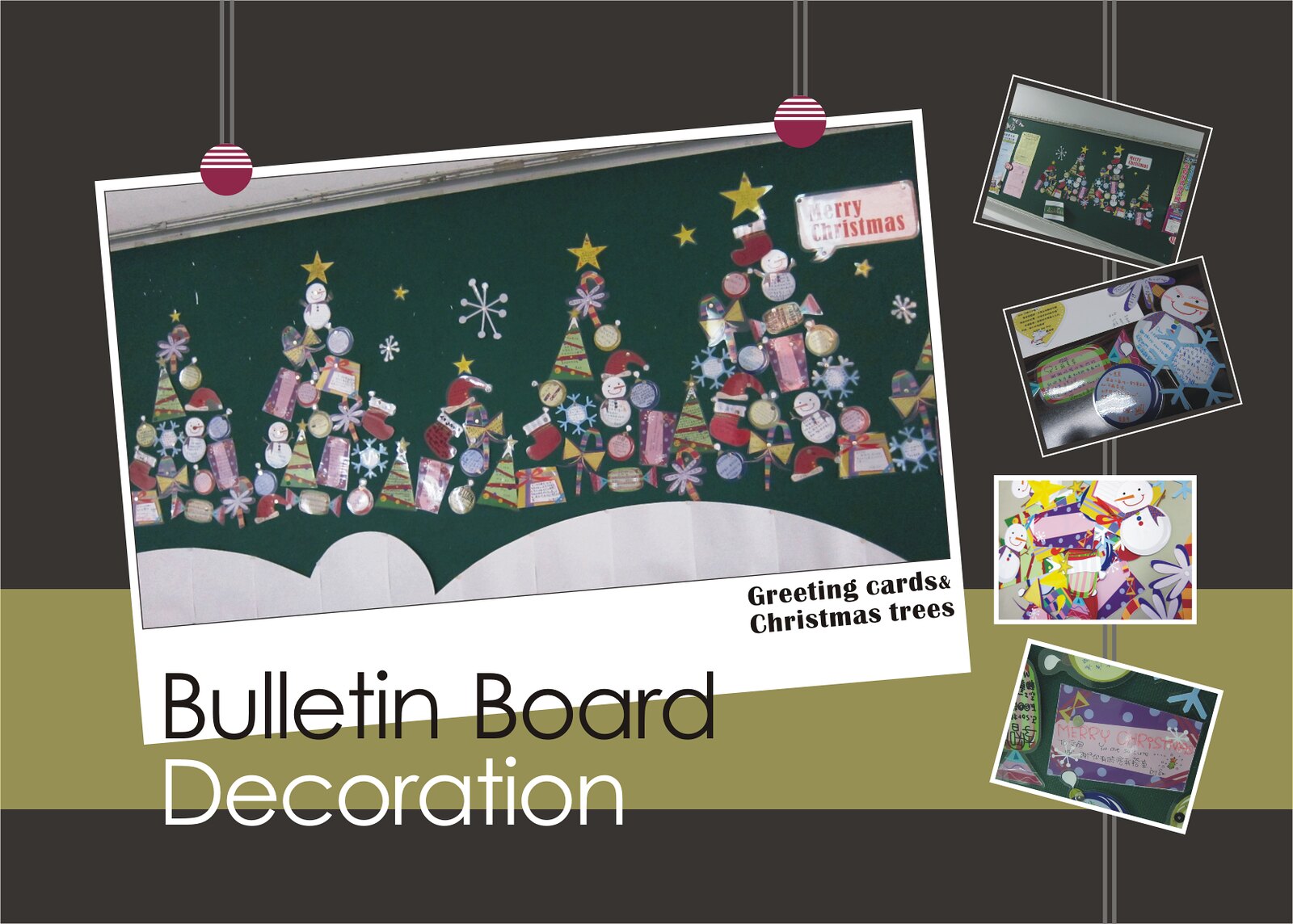This is an advertisement-like image with a festive, detailed design. The background features a dark emerald green color, contributing to its Christmas theme. Dominating the center of the image is a slightly tilted postcard, showcasing a collage of Christmas gifts, greeting cards, and vibrant Christmas trees, each topped with a gold star. There are five trees in total, adorned with various Christmas-related decorations, including stockings, ornaments, and presents. Below this central postcard, the text "Bulletin Board Decoration" is prominently displayed. Towards the right-hand side of the image, a series of smaller, slightly angled images are arranged in a zigzag pattern. These include a picture of a bulletin board with Christmas trees, a greeting card, a snowman graphic, and a tag resembling one from a Christmas package. The overall composition conveys a rich, festive spirit perfect for the holiday season.